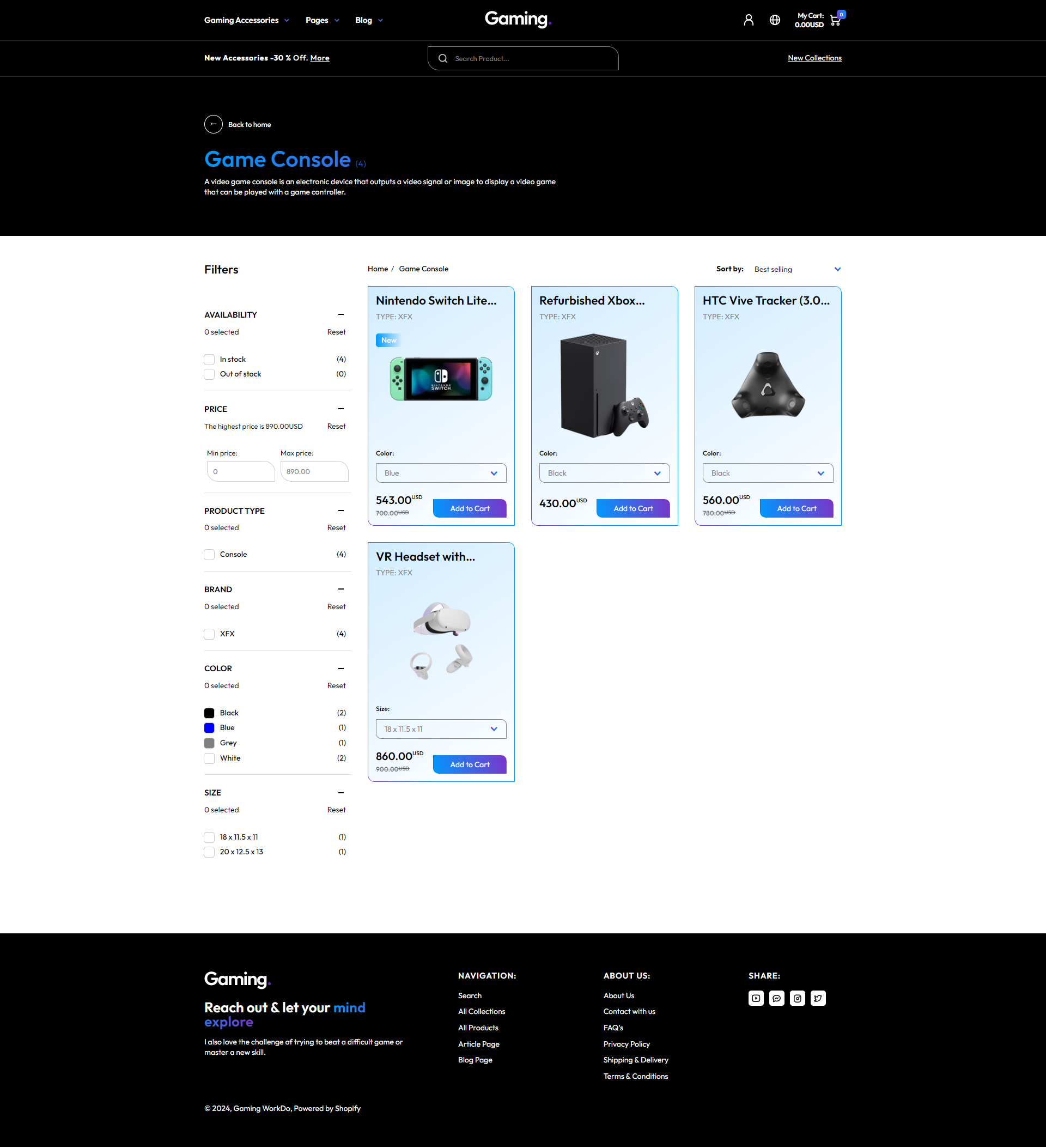The top portion of the interface is black, and the bottom part is equally black. It appears to be highly zoomed in, focusing on specific elements. At the very top, 'Game Aim' is prominently displayed, followed by a search bar beneath it. To the right of the search bar, there's an icon that likely represents a user profile.

Moving down and to the left, various game consoles are featured. First, we see the Nintendo Switch Lite, characterized by its blue Joy-Con controllers on either side. The Joy-Cons feature D-pad buttons, analog sticks, action buttons, a home button, and the Switch logo. The left Joy-Con is blue, while the right one is red.

Next to it is a refurbished Xbox Series X, which is essentially a tall rectangular box. It has the signature Xbox button, ventilation grilles on the top, and includes a controller with analog sticks and buttons.

Also displayed are HTC trackers, which are triangular in shape. Below the Nintendo Switch Lite is a VR headset, showcasing the front segment where the screens are located, along with the head straps. The VR controllers have circular rings designed for tracking purposes.